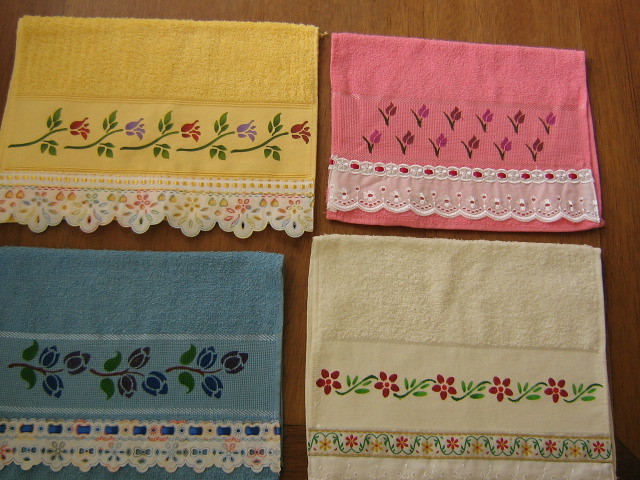The image depicts a bird's eye view of four neatly folded, old-fashioned cloths, each adorned with floral patterns and lace trimmings, laid out on a wooden surface. The top-left cloth is yellow terry fabric with a strip of yellow material, featuring a design of stitched red and purple flowers with green stems and leaves, bordered with intricately colored white lace. To its right, the pink terry cloth displays red and pink flowers with green stems, accented by a white lace border with pink dots. Below the yellow cloth, the blue terry fabric features dark blue flowers with green stems, framed by lace with satin blue stitching. Finally, the off-white terry cloth on the bottom right showcases five-petaled red flowers with green stems on white material, highlighted by a ribbon border with red flowers and colored squiggles. Each cloth exhibits meticulous detailing, resembling vintage hand towels or wash rags.